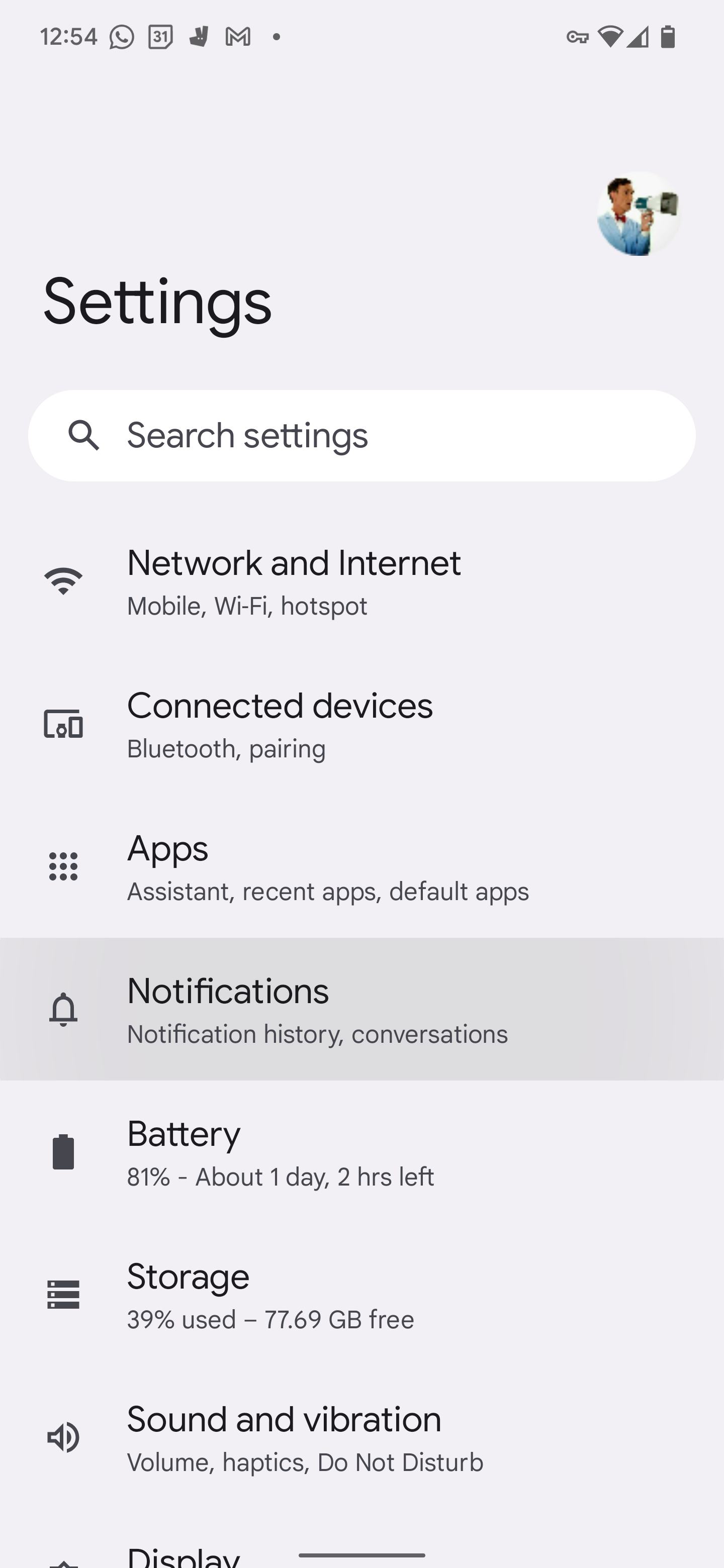This image showcases the settings screen of a cell phone, captured at 12:54. At the upper left corner, the current time is displayed, followed by a series of icons: the call bubble icon, the calendar icon, and the Gmail icon. On the upper right side, the screen displays a key icon, the Wi-Fi icon, the cell phone reception bars, and the battery icon. Positioned to the right of the screen's center is a round, speaker-like symbol, which appears to be a voice command or accessibility feature. Below this symbol, left-aligned, is the word "Settings".

Underneath the "Settings" title, a vertical list of options begins. It starts with a search bar labeled "Search settings". The first item in the list is "Network & Internet," which includes sub-options such as mobile, Wi-Fi, and hotspot. Following this, "Connected devices" is listed, featuring options for Bluetooth pairing. The next item is "Apps". The "Notifications" section, which appears to be selected, is listed below "Apps". Continuing down, we find "Battery", "Storage", and finally "Sound & Vibration". Each category is clearly delineated, providing a comprehensive view of the cell phone’s settings options.